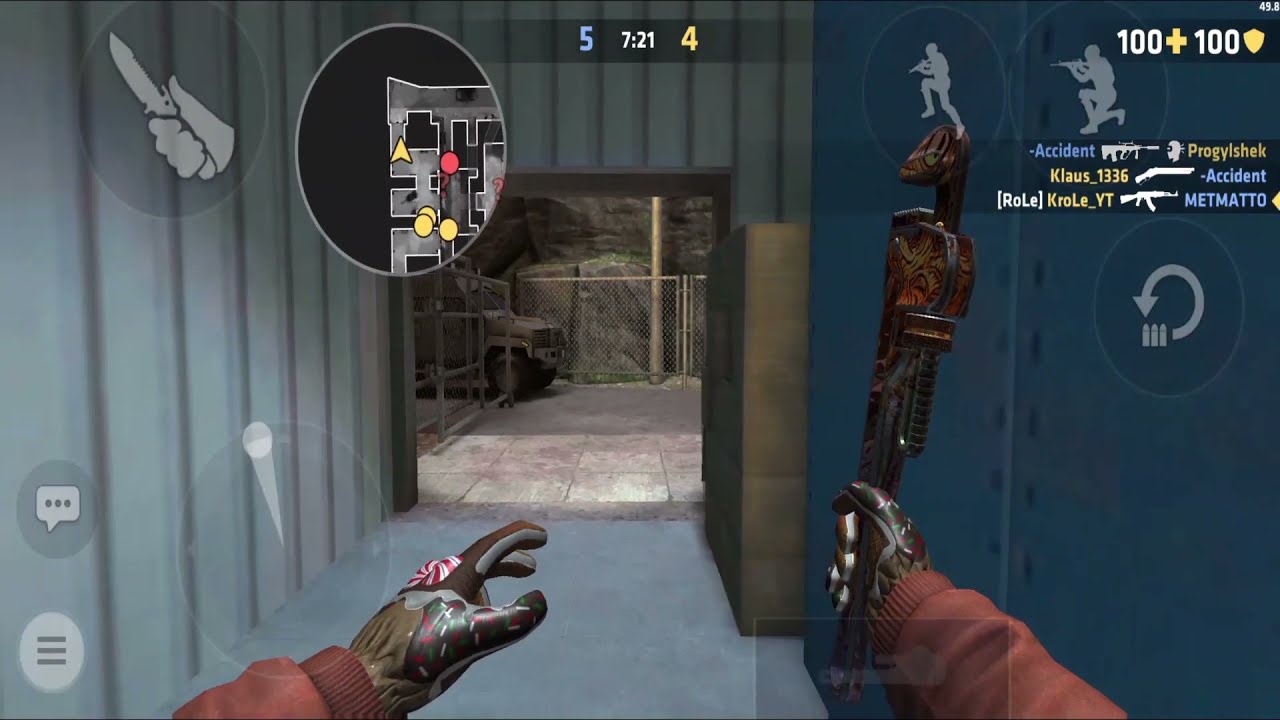The image is a screenshot from a first-person video game displayed in a horizontal rectangular format. The scene shows a hallway leading towards an open, large, thick brown door, through which a room with a white stone floor is visible. Inside this room, a truck can be seen to the left, near a gate, with a stone wall at the back. 

On the left-hand side of the screen is a wall with vertical panels and various icons: in the upper corner, an icon of a hand holding a knife, and in the lower corner, joystick controls, and menu buttons. In the middle, there is a mini-map displaying information about the game location and players.

The game's interface includes a scoreboard at the top center, showing a blue '5', yellow '4', and a time '7:21'. To the top right, health and shield indicators register as '100' each, accompanied by functional buttons for different player actions such as jumping, crouching, and reloading.

In the foreground, the primary character's arms extend into the image from the bottom, wearing red or maroon sleeves with green and white gloves resembling Christmas colors. The right hand, gloved and holding a decorated pipe wrench featuring a bird's head design, points forward. Surrounding the character, the hallway walls are blue steel, creating a factory-like environment. There are also various informational diagrams and icons throughout the screen, enhancing the immersive gaming experience.